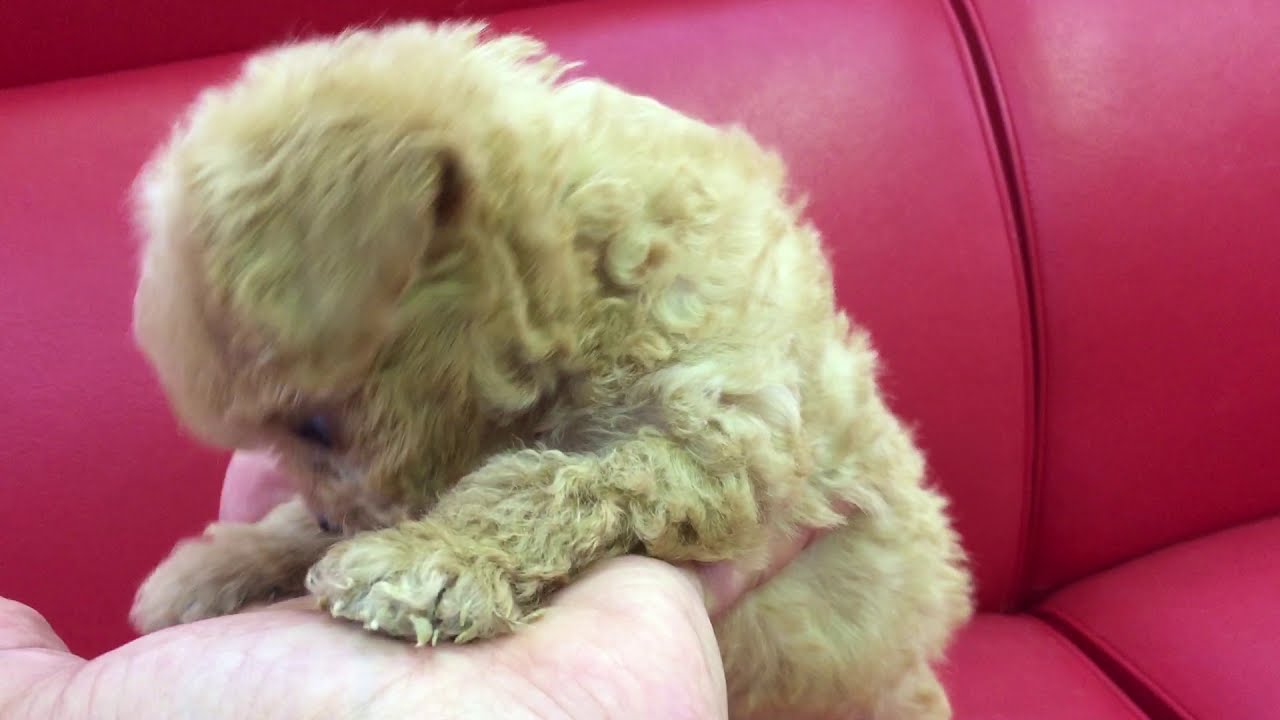This indoor photo features a small, curly-haired puppy with fluffy, light beige fur, almost a dirty blonde shade. The image is a close-up shot, slightly blurry as if the puppy was in motion, capturing the puppy's profile rather than a direct face view. The puppy is positioned in a light-skinned human hand, which is visible on the lower left side of the frame. The tiny dog appears to be attempting to climb up the hand, with its front paws resting on the hand and its rear end hanging just below it. The background of the image includes vibrant red chairs or a couch, adding a contrasting backdrop to the scene. The puppy's black eyes and tiny, curly frame make it an undeniably cute focal point.